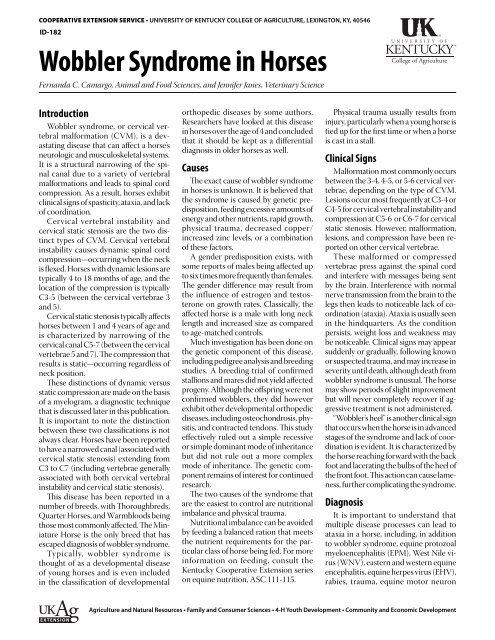The image depicts a vertically aligned rectangular snippet from a newspaper or magazine page, featuring detailed information about Wobbler Syndrome in horses. The background is plain white with no visible borders, measuring approximately four inches high by three inches wide. At the top of the page, the header in small black print reads, "Cooperative Extension Service, University of Kentucky College of Agriculture, Lexington, Kentucky, 40546," followed by "ID 182."

Prominently displayed in large bold black text below the header is the title, "Wobbler Syndrome in Horses." The upper right corner also features the text "UK, University of Kentucky College of Agriculture." The authors of the article, Fernanda C. Camargo of Animal and Food Sciences and Jennifer Janes of Veterinary Science, are listed immediately below the title.

The content on the page is organized into three justified-alignment columns of text. The first column, labeled "Introduction," provides an overview of the topic. The second column, titled "Causes," discusses the reasons behind the syndrome. The third column is split into two sections: "Clinical Signs" and "Diagnosis," detailing the symptoms and diagnostic procedures associated with Wobbler Syndrome.

A horizontal line separates the header from the main text. The footer of the page includes information about UKAG Extension, listing various departments such as Agricultural and Natural Resources, Family and Consumer Sciences, 4-H Youth Development, and Community and Economic Development.